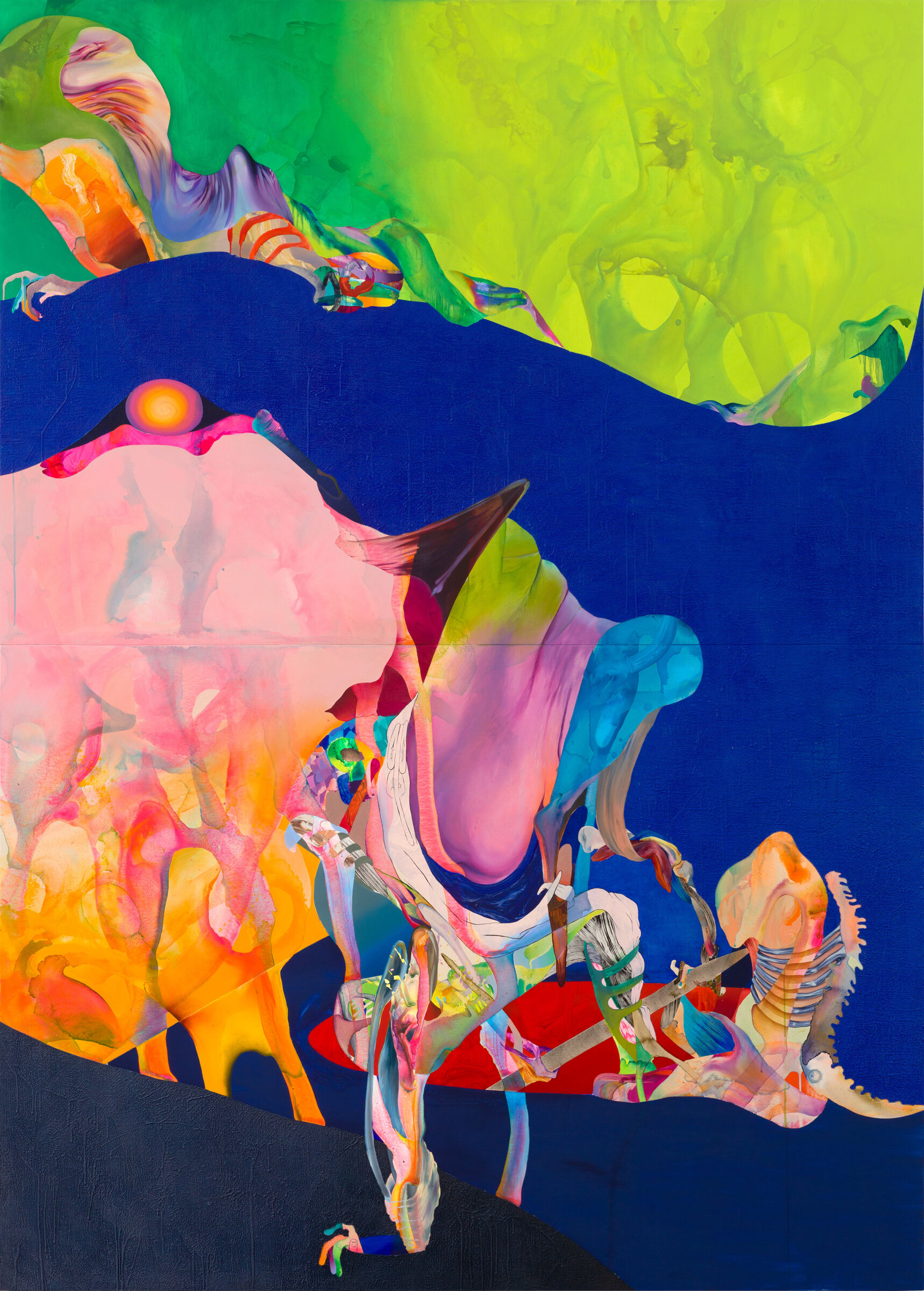The image is an intricate and very abstract painting that incorporates diverse colors and patterns, giving it a dynamic and complex appearance. In the top right-hand corner, a light neon green patch creates a smoky effect, blending into a darker green patch in the top left corner. Between these green areas, there is a striking juxtaposition of pink and purple designs. The middle portion of the painting transitions into a predominantly blue background, housing an array of eclectic and colorful elements. This central area displays a chaotic mix of pink, yellow, orange, and light blue hues with red and purple accents, forming amorphous and indistinct shapes that evoke a sense of confusion and abstraction. There is a green blob curling across the top part of the image, resembling slime, while in the lower regions, abstract forms suggest skeletal or hand-like shapes. A notable feature is a pink blob with yellow drips on the left side, juxtaposed by a contrasting light blue and red area. These colorful patches, patterns, and curves, rendered in a watercolor or acrylic medium, contribute to the painting's overall surreal and enigmatic aesthetic.